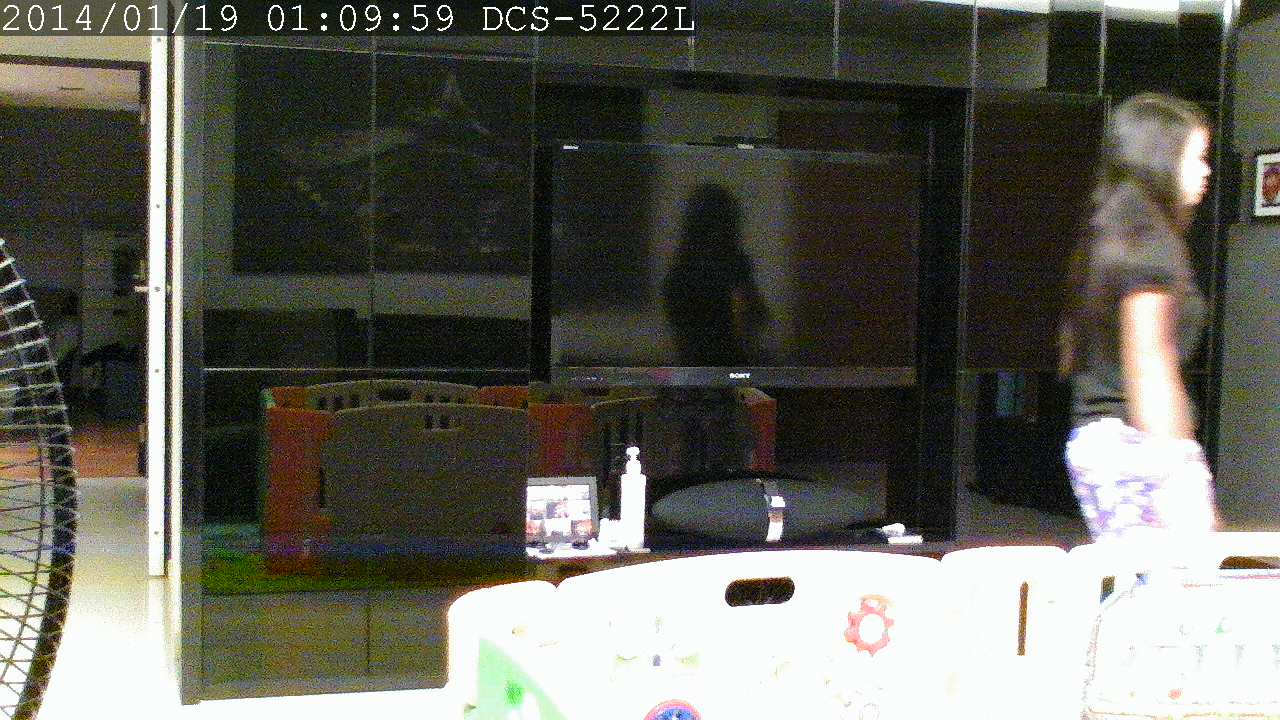A slightly blurry, rectangular image with a timestamp in white text at the top left corner reading "2014-01-19 01:09:59 DCS-5222L." On the right side of the image, a woman with black hair is captured in motion, moving towards the right. She is dressed in a black t-shirt. Centrally located behind her, there is a television with a black screen and a matching black frame.